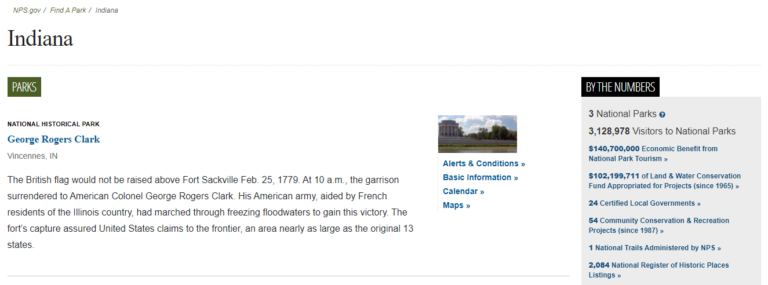This is a screenshot of a website section from nps.gov/findapark/indiana. The webpage has a white background with black text and blue accent text. At the top, the header reads "Indiana," separated by a gray line from the rest of the content. Below the header, there's a green button labeled "Parks" in white text.

The main text section highlights the National Historical Park, specifically George Rogers Clark National Historical Park in Indiana. It recounts a significant historical event: on February 25, 1779, at 10 a.m., the British flag was not raised above Fort Sackville as the garrison surrendered to American Colonel George Rogers Clark. Clark’s American army, aided by French residents of Illinois County, had marched through freezing floodwaters to seize this victory. The capture of the fort secured the United States' claim to the frontier, an area almost as large as the original 13 states.

To the right of this text, there is a small image, presumably of the park, although the details are unclear due to its size. Below the image, there are links labeled "Alerts & Conditions," "Basic Information," "Calendars & Maps," and a further section titled “By the Numbers” in a black box with white text. This section provides various statistics, highlighting the scale and impact of the National Park Service's work, including the number of national parks, certified local governments, and national trails managed by the NPS.